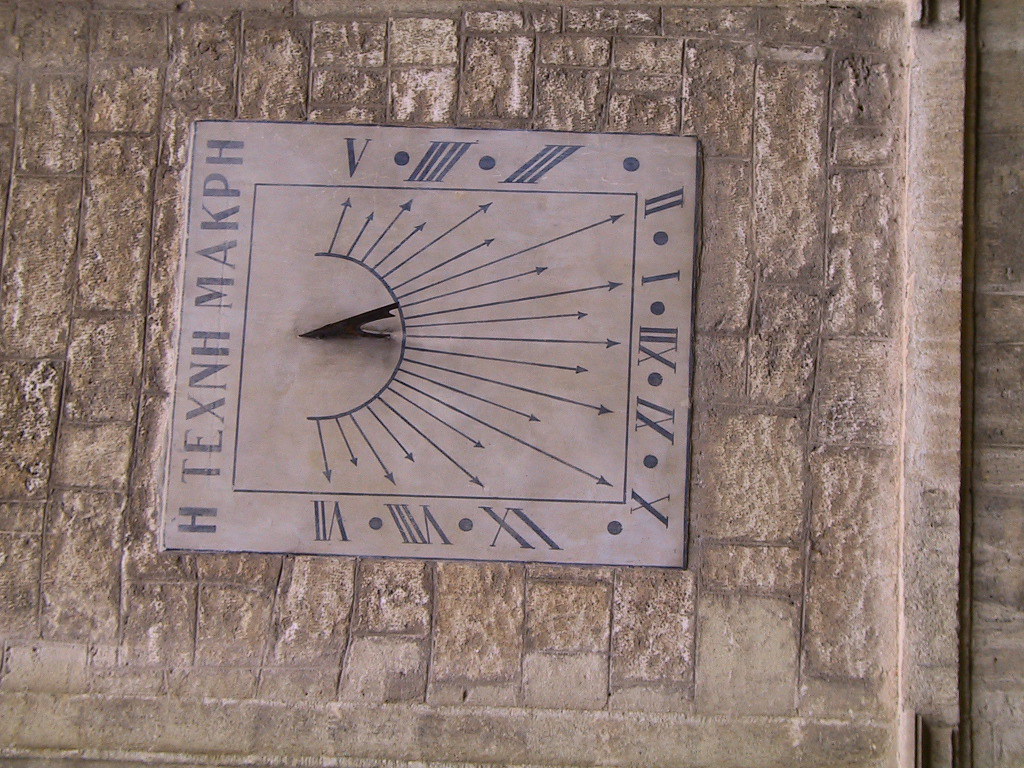This image showcases a square sundial made of a light tan, smooth stone, situated on a coarse, tan brick wall. The sundial features Roman numerals in black, arranged along the top and sides to indicate the time, with smaller arrows pointing to these numerals. The sundial’s design includes a semicircle with arrows pointing in various directions, offset to the left. A raised portion in the sundial casts a shadow horizontally to the right. Along the left-hand side of the sundial, vertically written, are the letters ‘H TEXNH MAKPH’. The mortar between the rectangular, square, and horizontal bricks surrounding the sundial is a darker gray-brown, adding contrast to the sandy tones of the entire background.